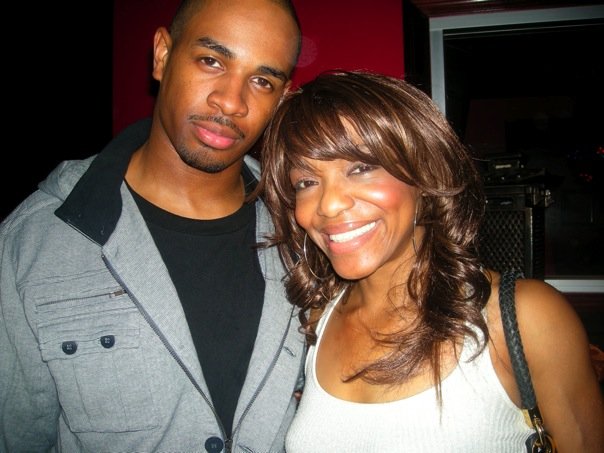The photograph features two individuals of African descent standing side by side against a red wall backdrop, with a dark window framed in black visible on the right side. On the left is a bald man with a short goatee, wearing a black t-shirt layered under a light gray zip-up jacket. He strikes a posed stance with a serious expression, slightly tilting his head towards the camera. To his right stands a woman with long, dark brown hair featuring bangs, and a glowing smile on her face. She is dressed in a white tank top and accessorized with large hoop earrings and makeup. She carries a black purse over one shoulder and the flash of the camera reflects brightly off her face, enhancing her joyful expression. The overall imagery suggests a moment that is both intimate and vividly captured due to the flash photography.